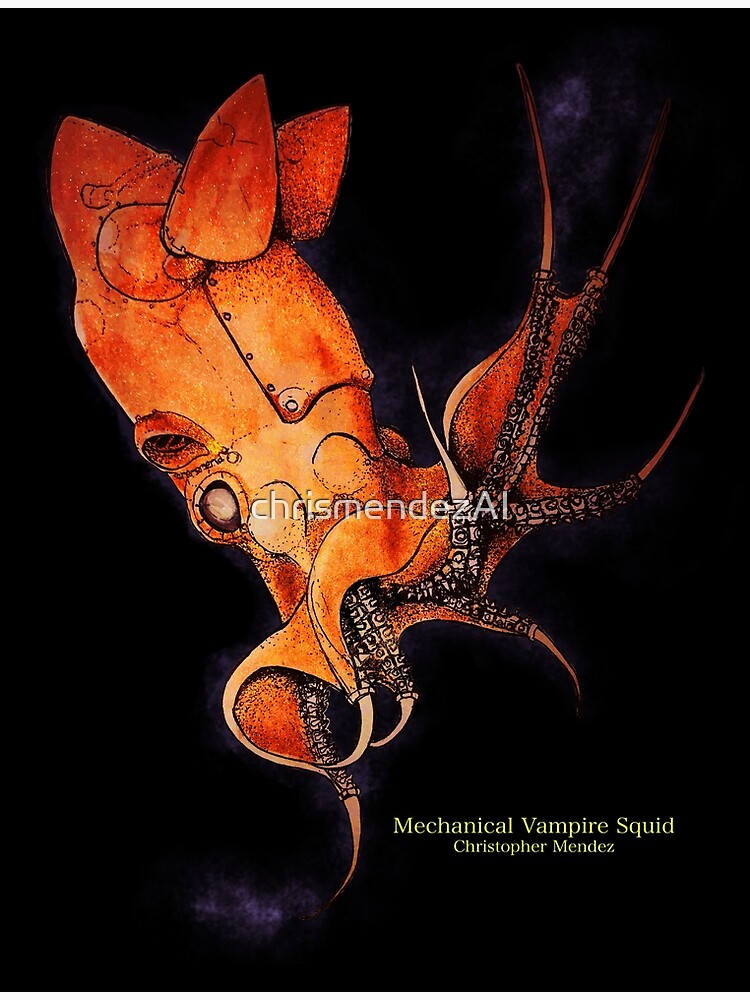The poster features a detailed and striking drawing of a mechanical vampire squid against a predominantly black background. The squid itself is primarily in hues of red and orange, with its tentacles showcasing a gradient to gray and black at the ends. The tentacles are decorated with intricate details including small suction cups and sharp, pink claws. The mechanical elements of the squid, such as its suckers fashioned out of chain links and bolts holding parts together, add a unique artistic flair. The lower right corner of the image prominently displays the text "Mechanical Vampire Squid" followed by "Christopher Mendez" in yellow letters. Across the center, a semi-transparent watermark reads "Chris Mendez AI" in white, signifying the creator and the innovative nature of the artwork. The overall image stands out with its clear depiction and vivid details.